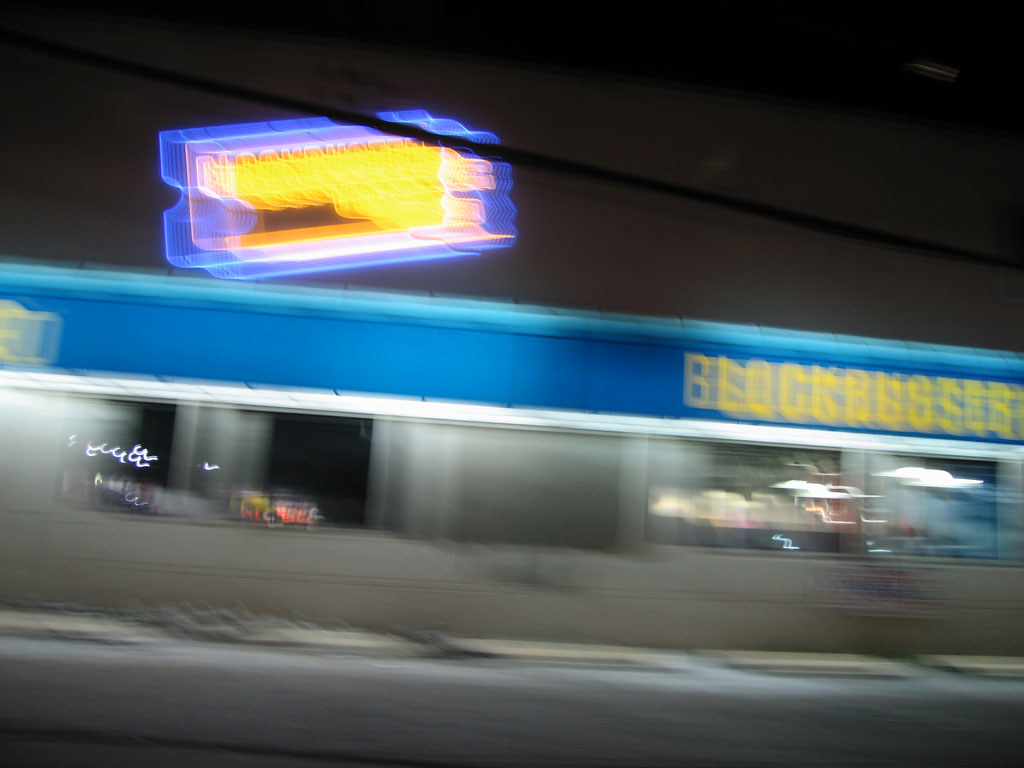The photograph, likely taken from a moving vehicle, captures a nighttime scene with a noticeable motion blur. The sky is an inky black, emphasizing the neon sign that dominates the image. This rectangular neon sign sits atop a building, glowing intensely with bright blue and yellow hues, although the text is unreadable due to the blur. Below the sign, the top of the building is illuminated in vibrant blue, with the word "Blockbuster" spelled out in gold, though slightly blurred but still legible. Beneath this, a thin white line runs horizontally across the building, just above a row of five windows that reflect light faintly. Below these windows, the building transitions into a gray section, giving way to what appears to be a sidewalk. Adding to the mystique of the image, small, white, 'W'-shaped lines appear on the left side of the building, while on the right, solid-shaped white "clouds" and other indistinct shapes hover, leaving one to wonder if these elements were a product of artificial intelligence enhancement.